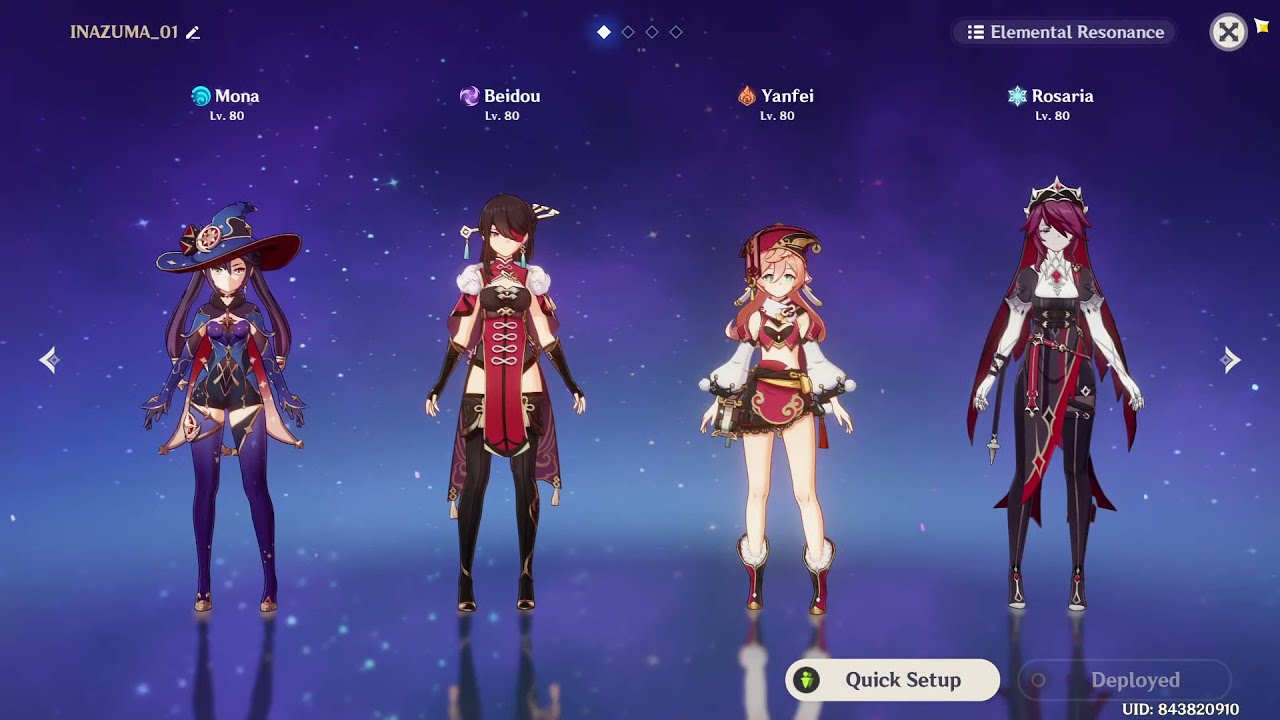The image appears to be a screenshot from the video game "Genshin Impact," featuring four anime-style female characters standing against a galactic-themed background dominated by purple and blue hues with scattered star-like elements. From left to right, the characters are:

1. **Mona**: She is adorned in a blue and red wizard hat paired with long sleeves, a corset-like top, and purple stockings. Her outfit includes high heels and possibly two ribbons or pigtails at the back.
2. **Beidou**: She has brown hair and sports a pirate-inspired look, with a red top, high black leggings, and high heels. She accessorizes with a single dangly earring.
3. **Yanfei**: She is depicted with pink hair and a short, skimpy outfit. Yanfei wears a small hat with a coin hanging off it, a white top, red skirt, and boots.
4. **Rosaria**: She has long, red hair and a gothic style outfit, including a black blouse, a vest, black leggings, full-length pants, and a distinctive necklace with a large red gem.

The game's interface displays "Elemental Resonance" in the top right corner and "Quick Setup" along with "Deploy" tabs in the bottom right corner, with "Quick Setup" being highlighted. The overall presentation suggests a celestial or starry night backdrop, creating an immersive fantasy setting for the characters.